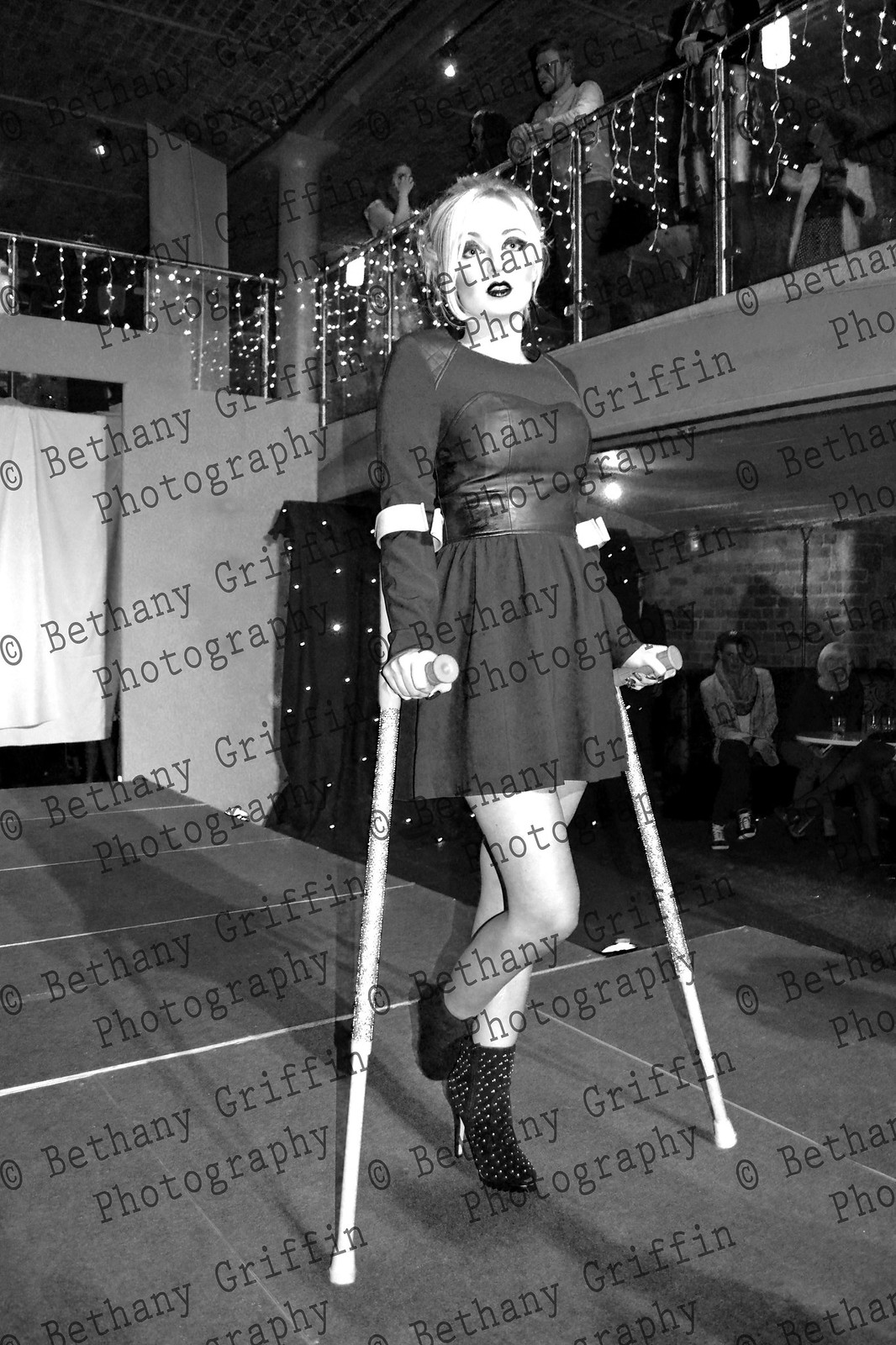In this detailed black-and-white photo by Bethany Griffin Photography, a woman is confidently walking down a T-shaped runway using crutches. Her light-colored hair and lipstick frame her determined expression as she models a black dress that reaches her thighs, paired with striking black boots adorned with silver studs. The room, which has two floors, is filled with spectators; on the bottom floor, people sit at tables with wine glasses, attentively watching the runway. Above, on the second floor, more attendees lean against a metal railing adorned with string lights, adding a festive ambiance. The stage, covered in fabric, features contrasting black and white tiles. The woman's left leg, bent at the knee, suggests she may be missing part of her foot, which is emphasized by her use of crutches wrapped around her elbows for support. The venue's thoughtful design and lighting highlight the significance of the event, creating a powerful and inspiring visual narrative.